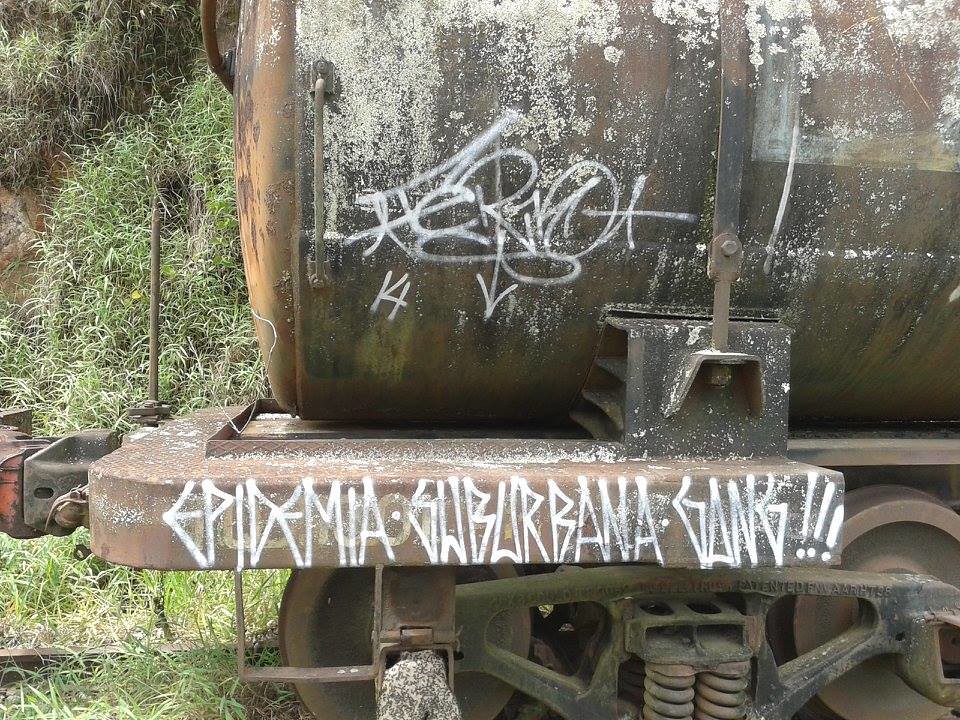The image showcases an abandoned and heavily rusted railway steam engine, depicted in a color photograph. The cylindrical tank, presumably a pressure vessel, is the focal point, riddled with rust presenting a palette of brown and orange hues. Rust extends to all visible parts, including the wheels, undercarriage, and the support springs, highlighting the engine’s disuse. Intricate details such as the exposed springs beside the wheels and unintelligible words etched across the axle can be seen. One legible word, "patented," stands out. 

Adorning the rusty surface is white graffiti, notably "Epidemia Surbana Gang" accompanied by an arrow pointing down and the number “14”. This graffiti, alongside patches of whitish residue, suggests long-term exposure to harsh elements. The disarrayed state of the engine is accentuated by a backdrop of long, patchy grass, and distant hills covered with more grass and trees. This setting amplifies the overarching sense of abandonment, further evidenced by white corroded spots on the tank car and graffiti splashed across its surfaces. The grass around the engine is overgrown, encapsulating the forlorn state of this once operational steam locomotive.